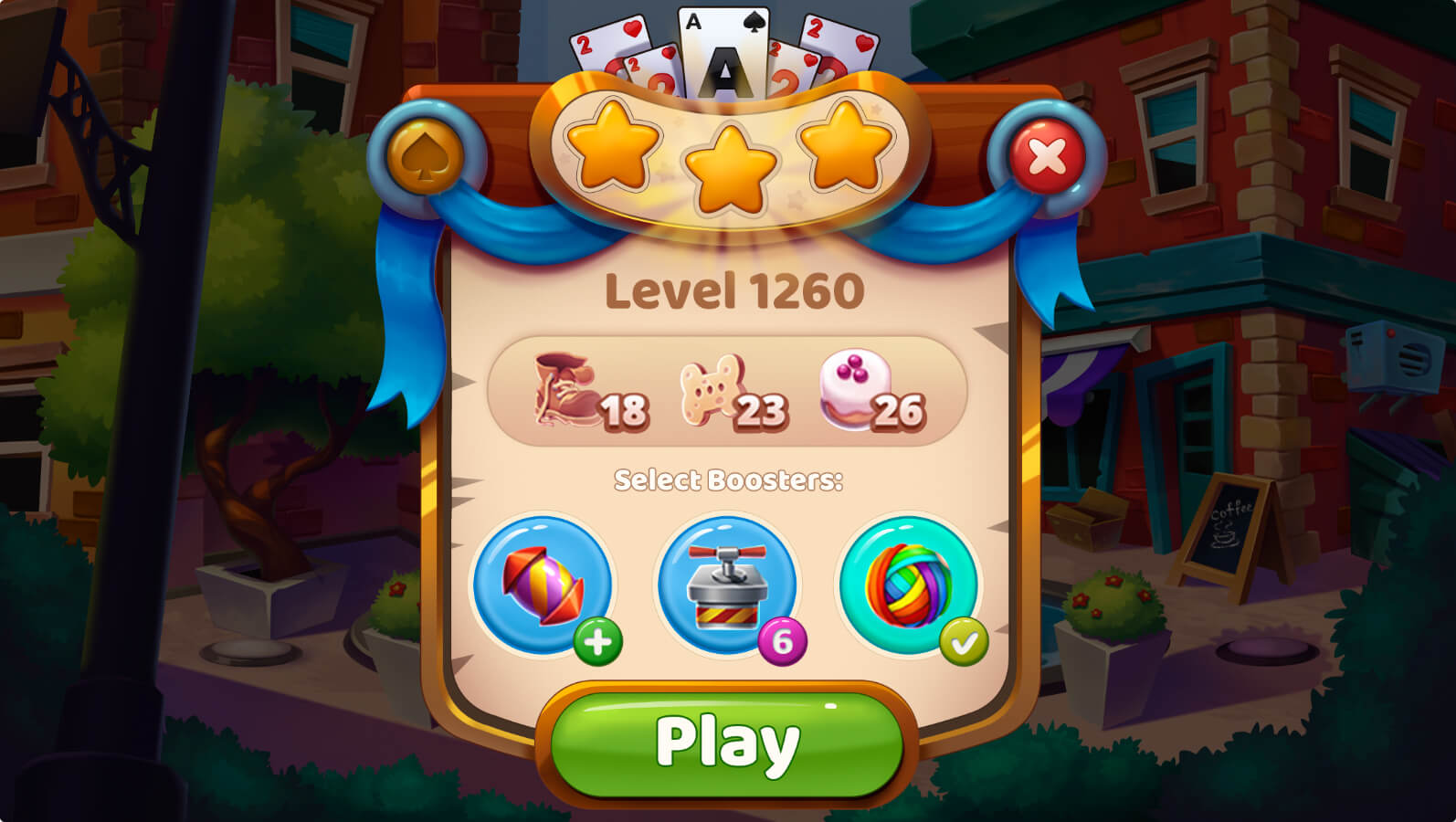The screen capture showcases gameplay from a vibrant, visually detailed game. In the background, there's a collection of brick buildings, some distinctly red and others with an orange hue, adding to the urban atmosphere. A metal post can be seen off to the side, contributing to the scene’s structural elements. Adding a touch of nature, there's a green tree planted in a pot alongside a flowering bush with red blossoms, also in a pot. A silver air conditioning unit is attached to one of the brick buildings, enhancing the realism.

Foreground elements include several cardboard boxes placed at the bottom of the scene. A green play button with white text is prominently displayed, indicating an interactive element. Among various colorful icons, a festive funfetti popper decorated in red, gold, and purple is placed on a blue circle, catching the eye. Another blue circle holds a silver, red, and yellow detonator icon with a purple-and-white '6' overlay.

Near a turquoise circle, there is a vibrant ball of yarn in a spectrum of colors—red, orange, yellow, blue, purple, and green—marked with a green checkmark. Above this, more icons are visible: a shoe labeled '18,' a dog bone with '23,' and a donut-like object decorated with white frosting and purple pearls labeled '26.' A blue ribbon banner, a red X, and a gold-colored spade icon add to the array of symbols.

At the top of the image, three gold stars highlight a scoring or achievement element, accompanied by playing cards featuring a two of hearts and an ace of spades. These details are captured in a high-quality, sharp, and vivid image.